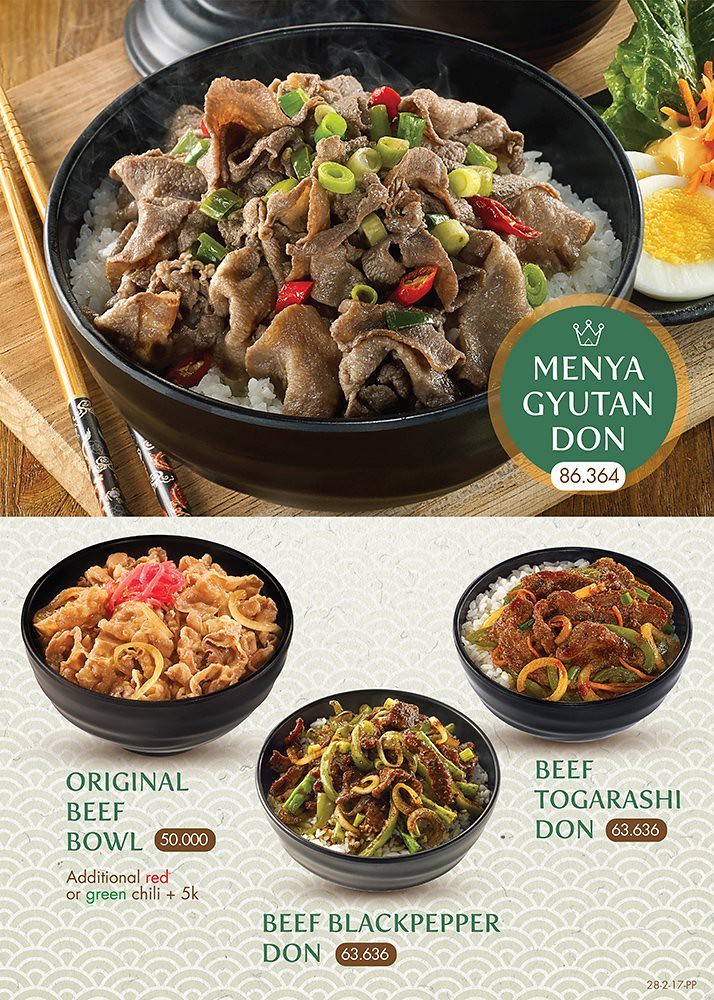The image depicts a detailed menu featuring several enticing bowls of food, emphasizing Japanese cuisine with elements such as chopsticks and vibrant ingredients. The top half of the image showcases a steaming black bowl filled with white rice topped with generously portioned meat, finely chopped spring onions, and chilies. Adjacent to the bowl are a set of artistically painted wooden chopsticks resting on a wooden surface. A side dish with grated carrot and a cooked egg is placed to the right, and the lid of the bowl hovers at the top edge of the scene. Overlapping this idyllic setup is a golden-green circle with white text that reads "Menya, Gyuten, Don," accompanied by a white cylinder displaying the number "86.364."

The bottom half of the image highlights three more appetizing bowls, each with white rice and a variety of toppings. On the left is a black bowl with meat and grated onions or radish, labeled as the "Original Beef Bowl" priced at 50.000, with an optional addition of red or green chili for an extra 5K. The central bowl contains green and brown meat with additional brown vegetables on white rice, named "Beef Black Pepper Don" priced at 63.636. Lastly, the rightmost bowl features beef, white rice, and a mix of yellow and green vegetables, labeled "Beef Togarashi Don" and also priced at 63.636. The background of this section features an arched, geometric pattern further highlighting the aesthetic appeal of the presented dishes.